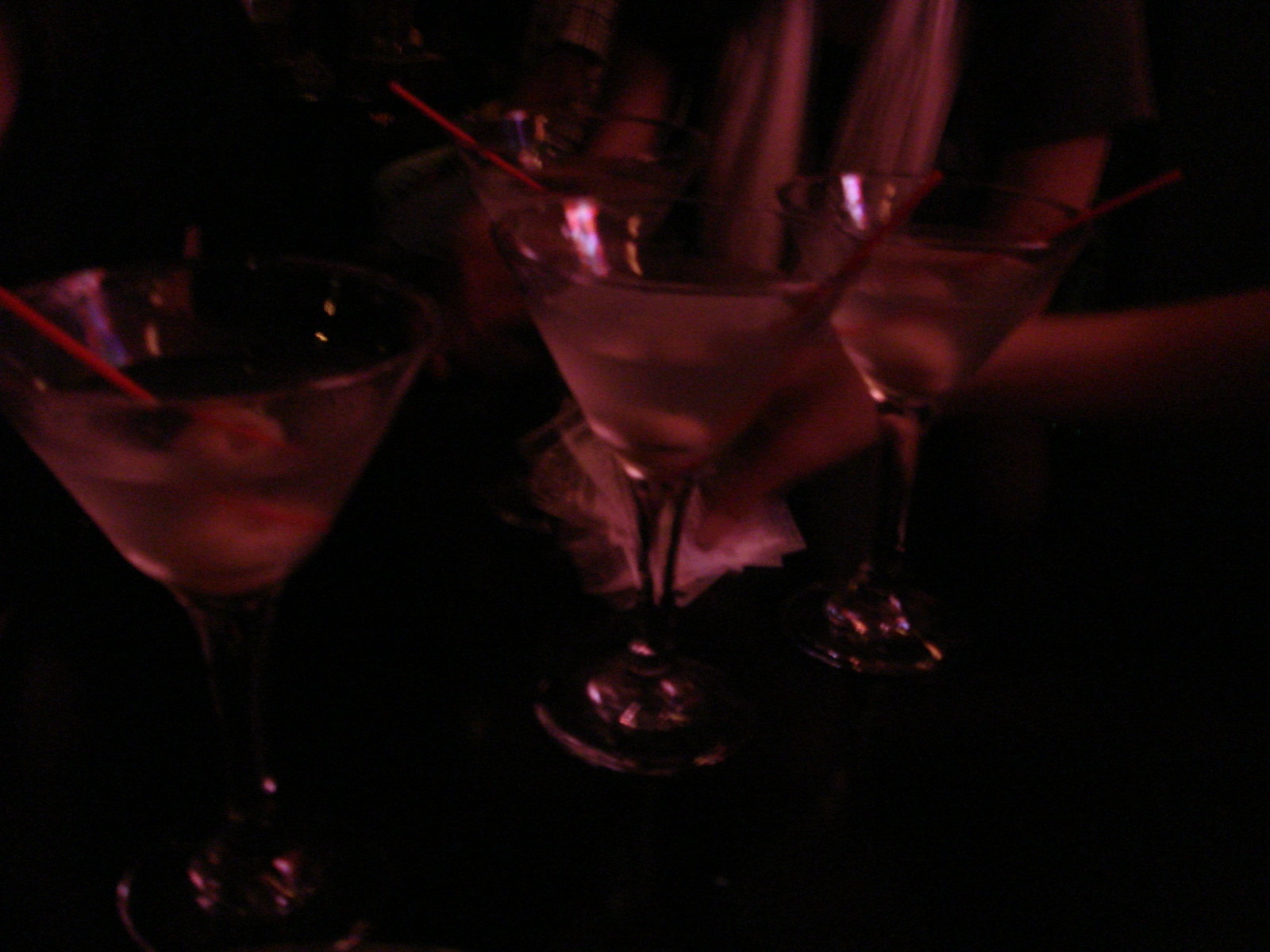This photograph, taken under dim lighting conditions, showcases three martini glasses lined up in a row on a dark countertop, likely at a bar. The image is heavily blurred, with a prominent red tint that bathes the entire scene in a reddish hue. Each of the martini glasses is clear, filled with a nearly transparent liquid that appears slightly cloudy. Skewered by thin red straws, pairs of green olives are submerged in each glass, with the straws extending out from the top. In the background, indistinct, blurry torsos of individuals can be made out, with one person appearing to wear a white scarf and possibly handling some form of paper currency. The overall blurriness and poor lighting make it challenging to discern precise details and colors, adding a mysterious atmosphere to the image.